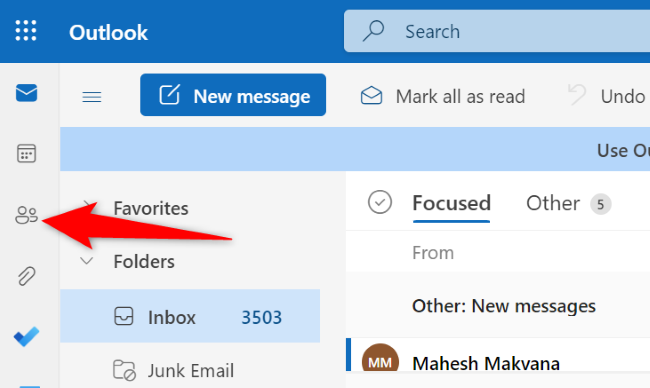Here is a detailed and cleaned-up caption for the described image:

---

The screenshot depicts a computer screen magnified for accessibility, showing an email client interface. The interface features a dark blue header bar across the top. On the leftmost side of this bar is a nine-dot grid icon, followed by the word "Outlook" in large text. To the right, there is a light blue, circular-edged rectangular search bar with a magnifying glass icon and the word "Search." 

Beneath the header, running vertically down the left side of the screen, is a light gray column containing five icons. A prominent red arrow points towards the middle icon, which depicts two people. 

At the top of the screen, beneath the primary dark blue header, there is a light gray secondary bar. This bar contains several elements, including a three-line hamburger menu icon, a New Message button in a dark blue rectangle, an envelope icon labeled Mark All as Read, and an Undo button.

Directly under the secondary toolbar, there is a light blue row that intersects the interface. The screen is then divided into two columns. The left column, shaded in light gray, lists navigational items such as Favorites, Folders, Inbox, and Email. The right column displays what appears to be the actual email messages.

---

This thorough caption reflects the specific visual elements and structure of the screen described.